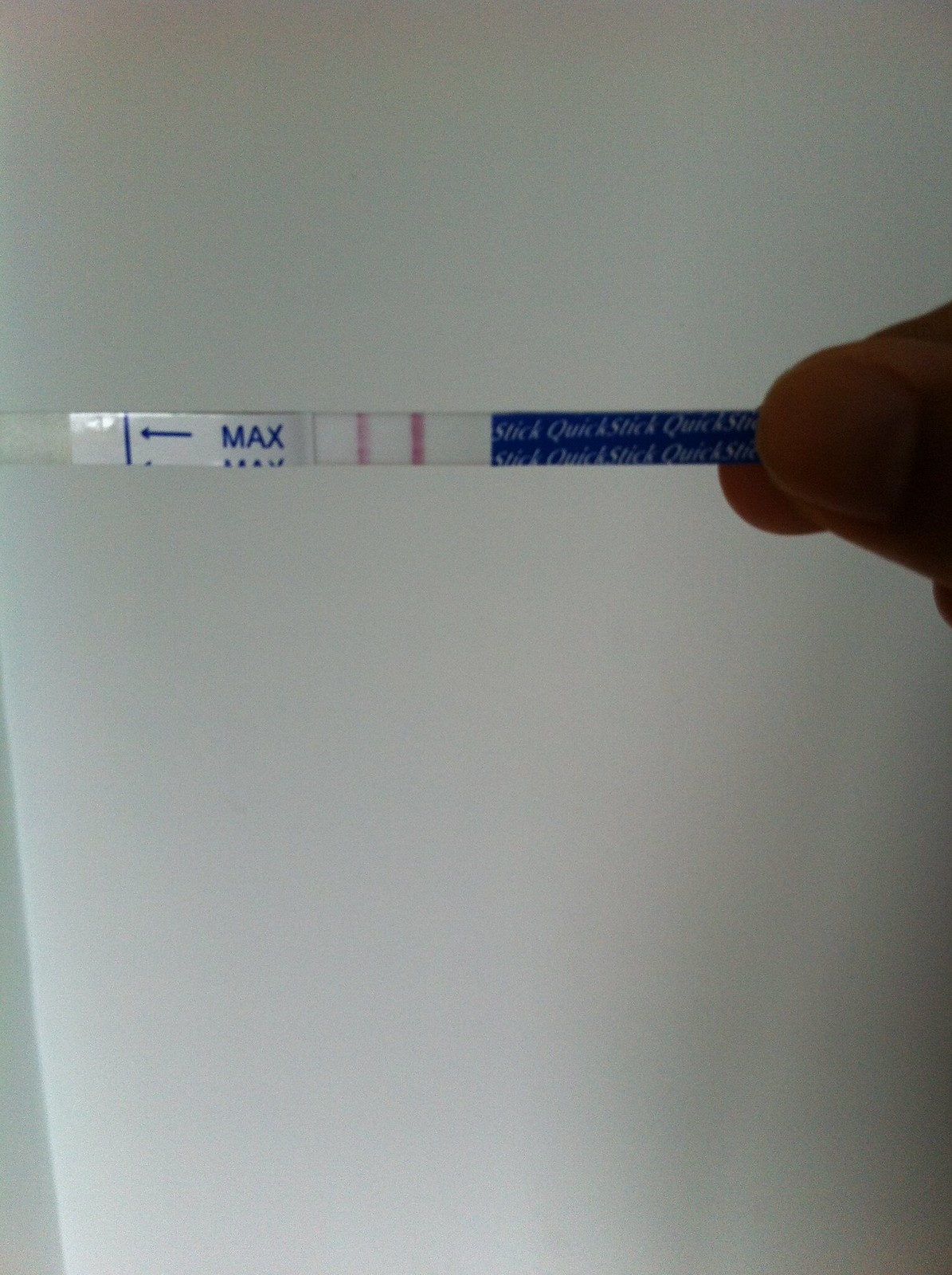The photograph depicts a minimalistic scene with a stark white background, slightly shaded on the bottom left and right edges. Emerging from the top right corner, a thumb and index finger are partially shadowed, obscuring the finer details of the skin. The fingers hold a small, clear plastic object, which resembles a pull tab. This object features a white sticker with a faint blue vertical line on the left side and an arrow pointing toward it. The text "MaxMAX" appears prominently in blue. Within the clear portion of the plastic, two red lines run parallel. Additionally, there is a blue section on the plastic, repetitively labeled with the phrase "stick quick stick quick stick." Overall, the image focuses on this small, detailed object against a plain background, highlighting its intricate design elements.